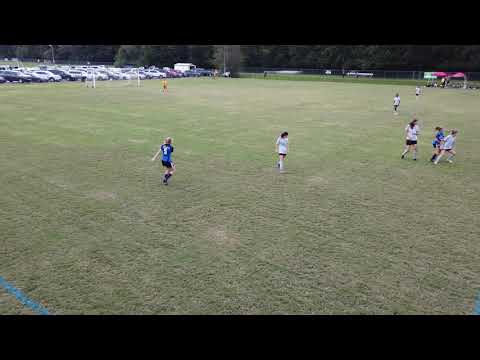The image captures a high-angle view, likely from bleachers or possibly from a drone, of a local girls' soccer game in progress on a large grassy field. The players appear to be teenage girls, with one team wearing blue jerseys with black stripes and black shorts, and the other team sporting white jerseys with red shorts. The action is concentrated in the middle of the field as the girls cluster around the ball. In the top left corner, a goalpost is visible with a line of parked cars behind it, suggesting a parking lot adjacent to the field. Additionally, there are a few people gathered under red canopy tents located on the right side of the image, likely where coaches or other participants convene. The background is framed by a row of trees, reinforcing the local and community feel of the scene. Despite the blurriness of the image, the details such as the players' attire and the setting indicate it is a children's soccer game taking place.